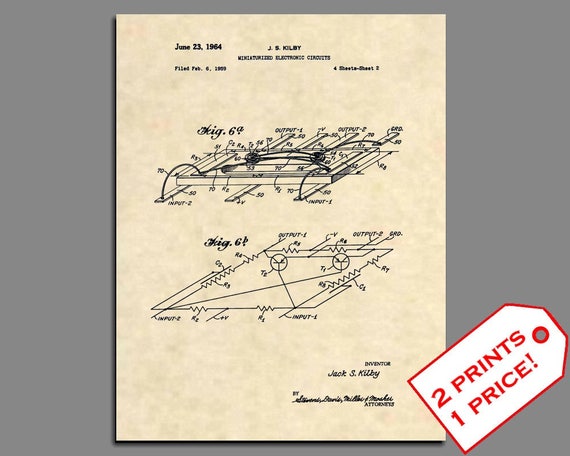This image showcases a square, gray background featuring a centered sheet of cream-colored parchment. The top of the parchment is marked with the date "June 23, 1964" and the name "J.S. Colby," followed by smaller, unreadable text and "filed February 6," though the full date is not discernible. The document contains detailed diagrams labeled "Figure 6A" and "Figure 6B," which depict both a physical layout and a schematic representation of an electronic device, complete with symbols for various components and interconnections. In the bottom right corner of the parchment, "Inventor Jack S. Kilby" is noted, along with an unreadable cursive name labeled as the attorney. Additionally, a price tag-like icon is displayed in the lower right-hand corner of the image, with a white tag outlined in red, containing bold red text that reads "Two Prints One Price!" This combination of elements seems to emphasize the availability of purchasing these detailed prints of Jack S. Kilby's invention diagrams.